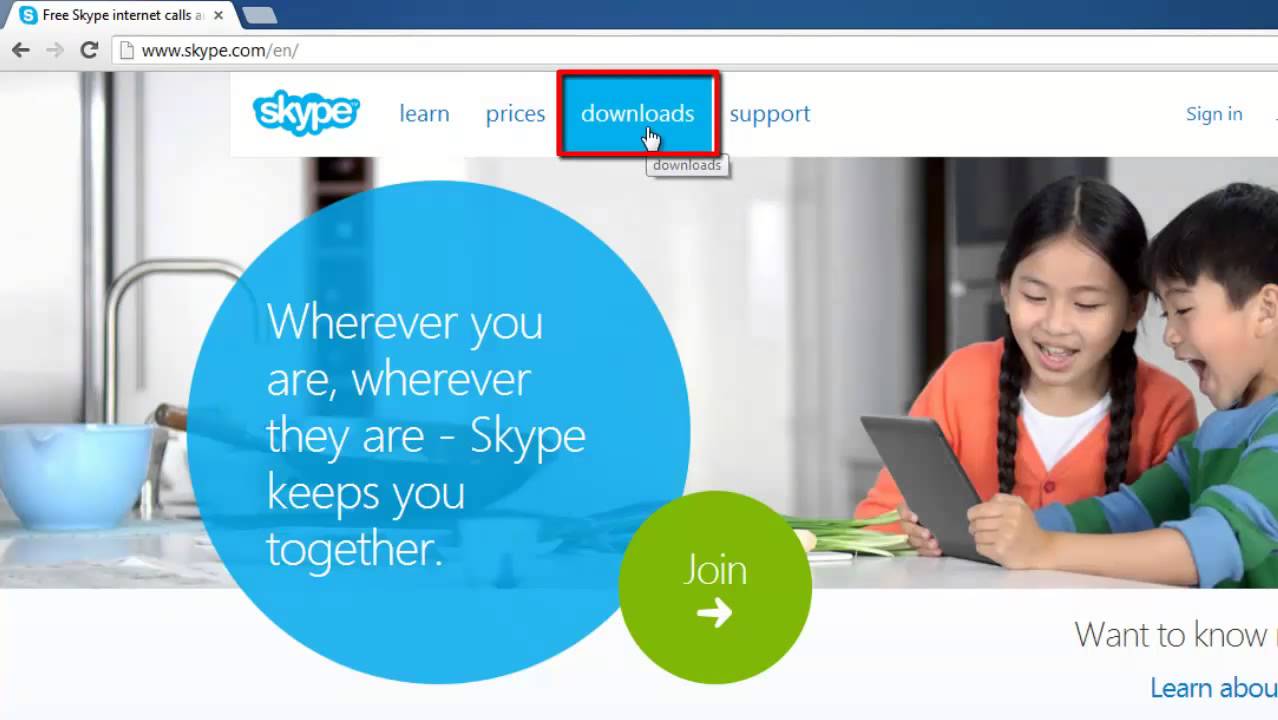In the top corner of the website, the text "Free Skype Internet Calls" is prominently displayed, with the URL www.skype.com/en visible. The website's main background features a cozy kitchen scene, complete with a small bar counter. On the counter, there is a sink with a wok and a pot beside it, along with a cutting board adorned with green onions, some of which are chopped, and a coffee mug. Dominating the center of the image are two children sitting at the counter, one around eight years old and the other roughly five to seven years old. The older child is a girl dressed in an orange sweater with buttons and a white shirt underneath, her hair styled in pigtails. She gazes intently at a tablet held by her younger brother, who wears a light blue and green striped shirt. Both children are visibly excited, smiling as they interact with the device. Adding context to their joy, a speech bubble on the screen reads, "Wherever you are, wherever they are, Skype keeps you together." Below this, a green bubble with the word "join" prompts viewers to learn about connecting with loved ones via Skype.